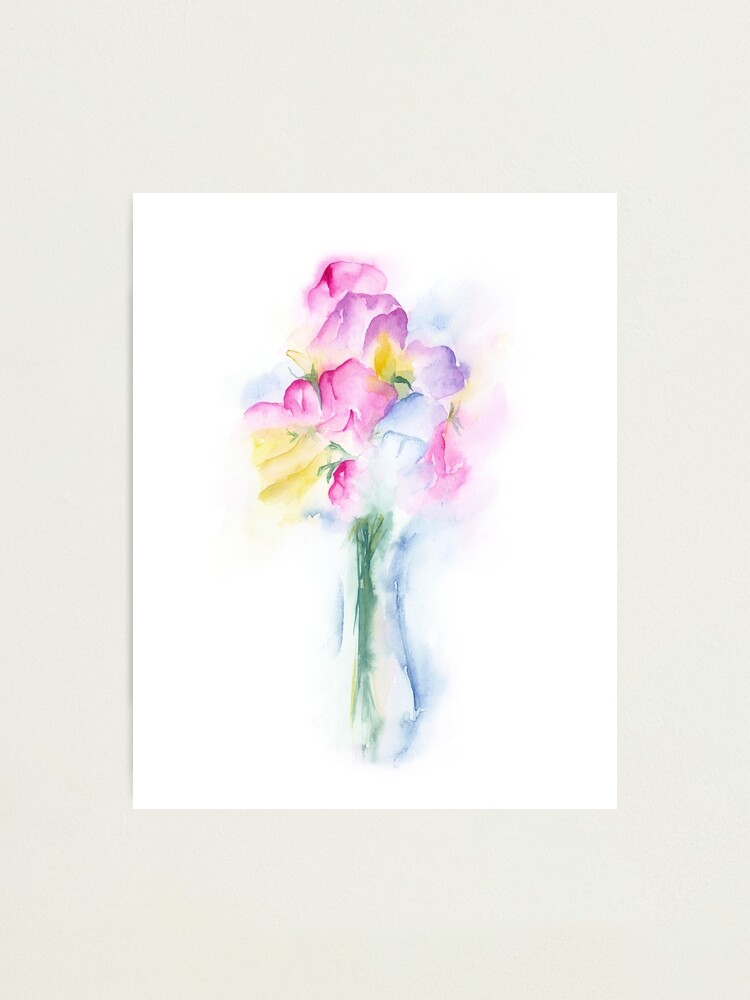The image showcases a delicate, abstract watercolor painting on white paper, set against a light gray background. The painting depicts a loosely defined bouquet of flowers in a tall, skinny, transparent vase, with a green-blue stem extending downwards. The bouquet itself is a delightful, clustered assortment of flowers in various hues, including pink, yellow, blue, and purple. The fluid, impressionistic style lends an ethereal quality to the piece, with the colors blending seamlessly. The painting is unsigned, without any border or frame, enhancing its simple, yet elegant charm, making it a perfect decorative piece for a home.